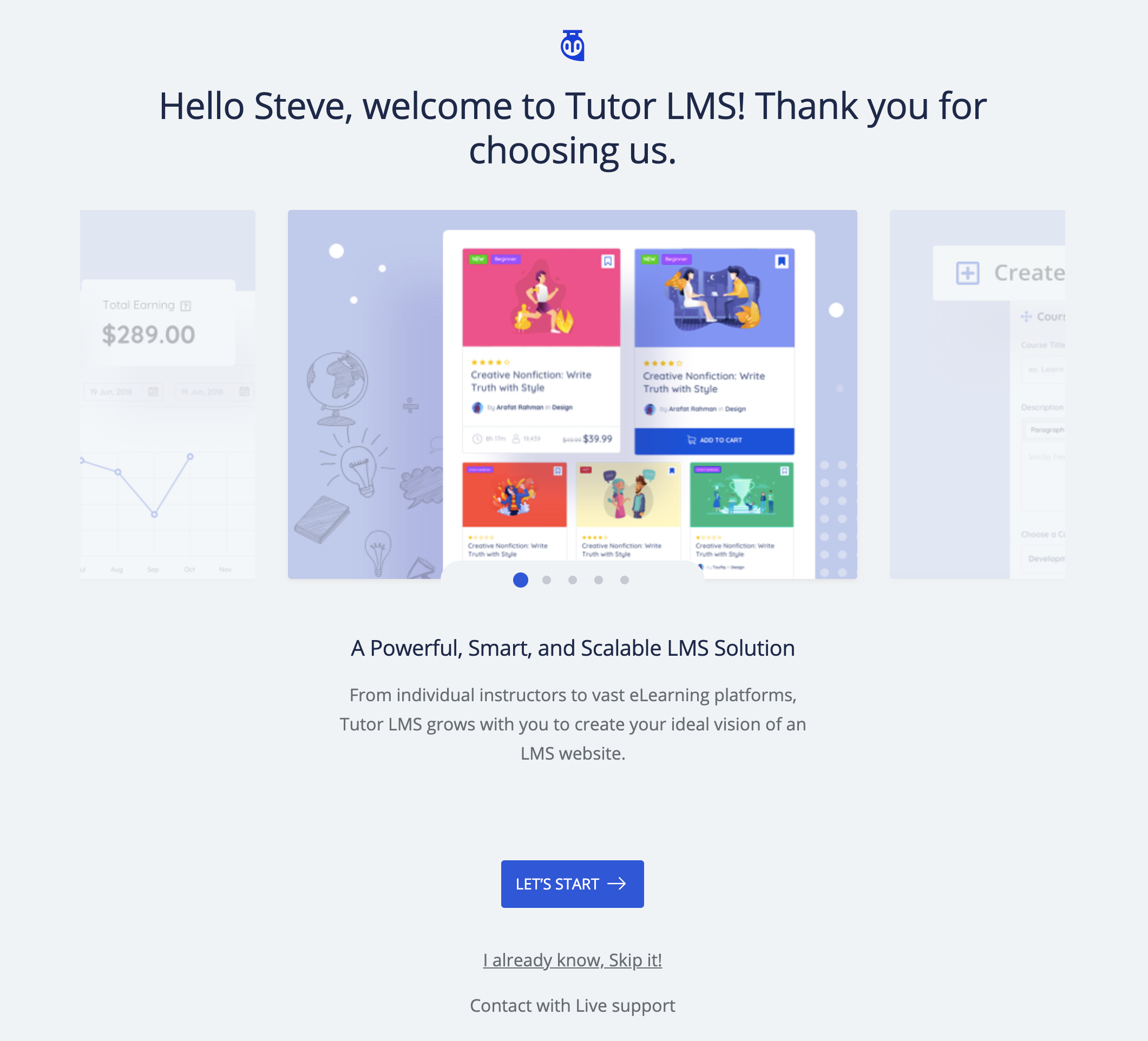The image is a website screenshot displaying an onboarding process for Tutor LMS. The primary color scheme is a dull light beige background with blue highlights. At the top of the screenshot, there's a small blue logo resembling an owl, accompanied by large black text that reads, "Hello, Steve, welcome to Tutor LMS! Thank you for choosing us." Below this text, three faded and transparent images flank a central, more vivid screenshot that features decorative illustrations like a globe, light bulb, book, and speech bubble. Underneath these images, text declares, "a powerful, smart, and scalable LMS solution."

Further down, smaller dark gray text elaborates, "From individual instructors to vast e-learning platforms, Tutor LMS grows with you to create your ideal vision of an LMS website." At the bottom center of the screenshot, a blue button with white text reads, "Let's start," accompanied by a right-pointing arrow. Below the button is an underlined gray link stating, "I already know, skip it," and a smaller text line mentioning, "contact with live support." The website also displays earnings, different curriculum choices, and a carousel indicator suggesting multiple pages. This comprehensive layout serves as an advertisement and onboarding guide for Tutor LMS, showcasing its capabilities and inviting users to begin their e-learning journey.